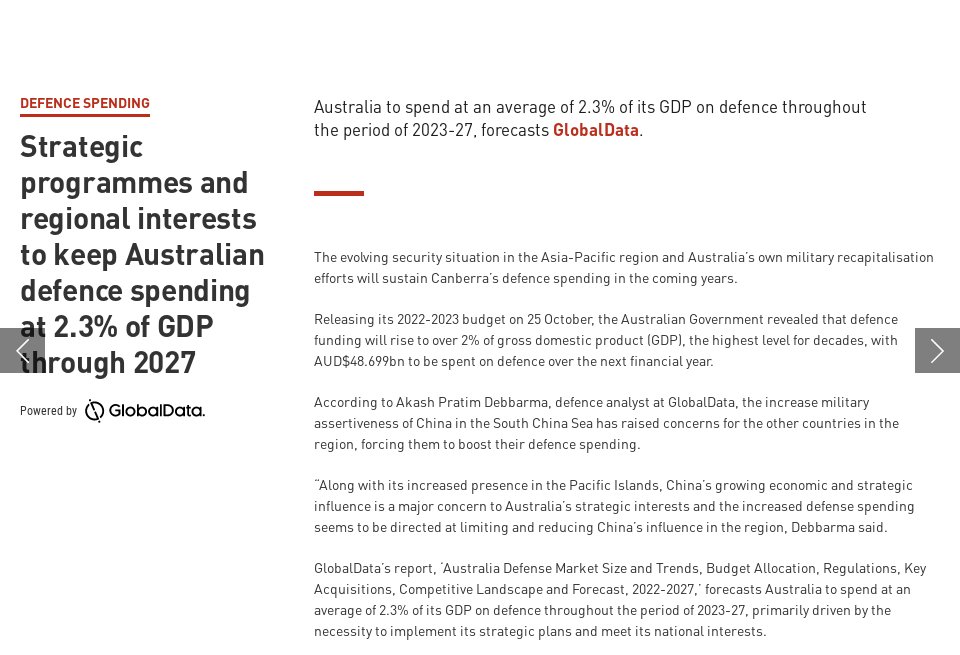This image, sourced from an article discussing Australian defense spending, features detailed graphic elements. Central to the image is a section that highlights "Strategic Programs" and "Regional Interests," emphasizing the commitment to keep Australia's defense spending at 2.3% of GDP through 2027. 

On the left side of the image, an arrow pointing to the left is positioned directly above the "2.3%" figure, drawing attention to the specific percentage. At the top of the image, the header "Defense Spending" is prominently displayed in red. 

To the right, the text reads "Australia to spend an average of 2.3% of its GDP on defense throughout the period of 2023 to 2027," followed by the source attribution "Forecast: Global Data," with "Global Data" in red. 

Additionally, there is a red line below this section, leading into a paragraph that states: "The evolving security situation in the Asia-Pacific region and Australia's own military recapitalization efforts will sustain Canberra's defense spending in the coming years. Releasing its 2022 to 2023 budget on October 25th, the Australian government revealed that defense funding will rise," with further details continuing down the page. 

The image provides a comprehensive visual breakdown of Australia's defense budget plans against the backdrop of regional security dynamics and internal military developments.